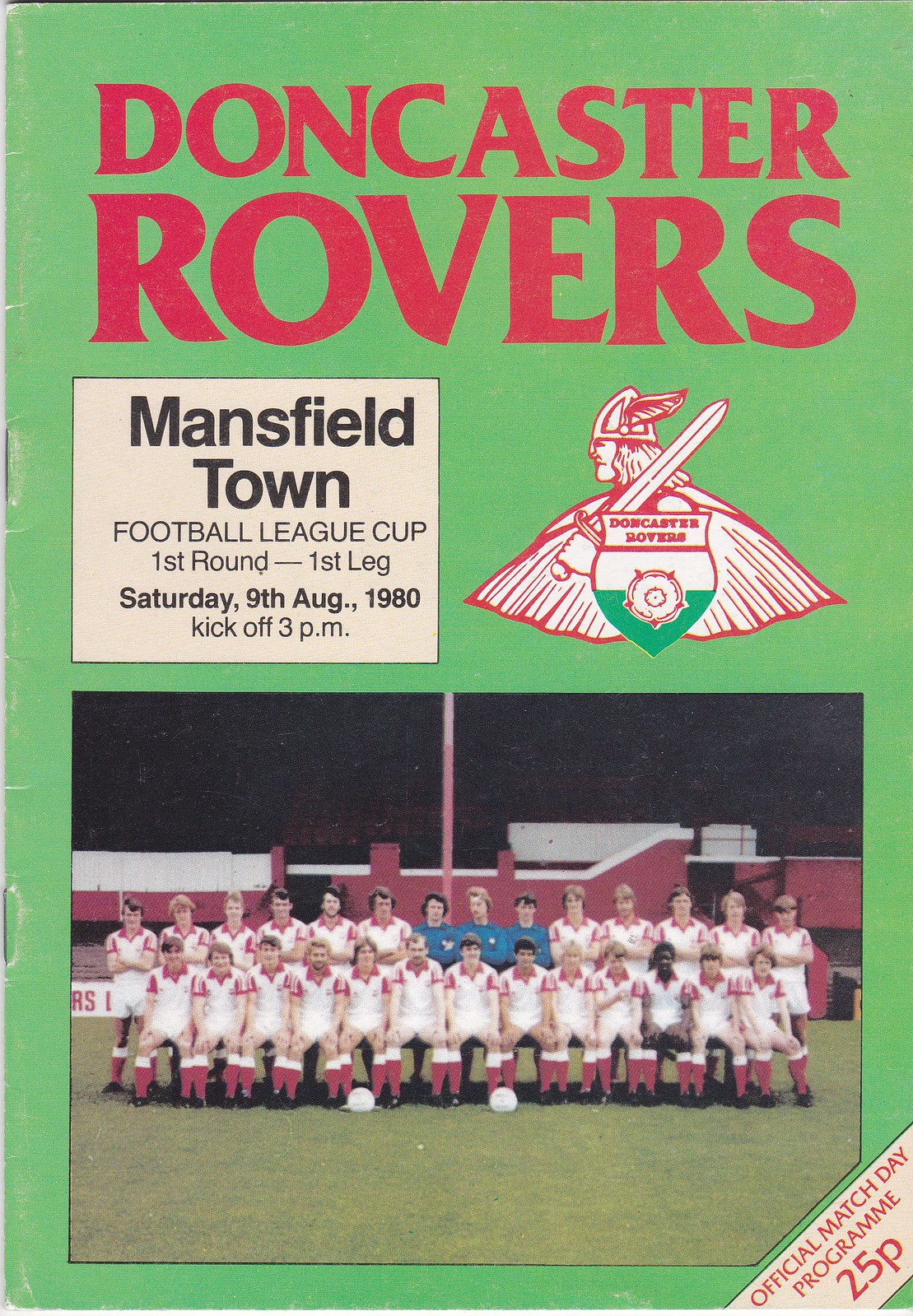The cover of the football program is predominantly green and features the title 'Doncaster Rovers' in bold red text at the top. Directly below that, a white square contains the text 'Mansfield Town' in black. This white box further includes details about the match: 'Football League Cup, First Round - First Leg,' and the date and kickoff time, 'Saturday 9 August 1980, Kickoff 3 p.m.' To the right of the white box, there's an emblem depicting a figure with a winged hat holding a sword, which likely includes the Doncaster Rovers' shield. Beneath these elements, a photograph of a football team shows two rows of players in white uniforms with red accents, along with three individuals in the middle of the back row wearing blue, possibly coaches. The background of the photo displays some buildings, while the foreground features two soccer balls on grass. Two staples are visible along the left edge of the cover. In the bottom right-hand corner, a diagonal band has text that reads, 'Official Match Day Program, 25p' in red. The overall design is detailed with the text at an angle and patterned green background.